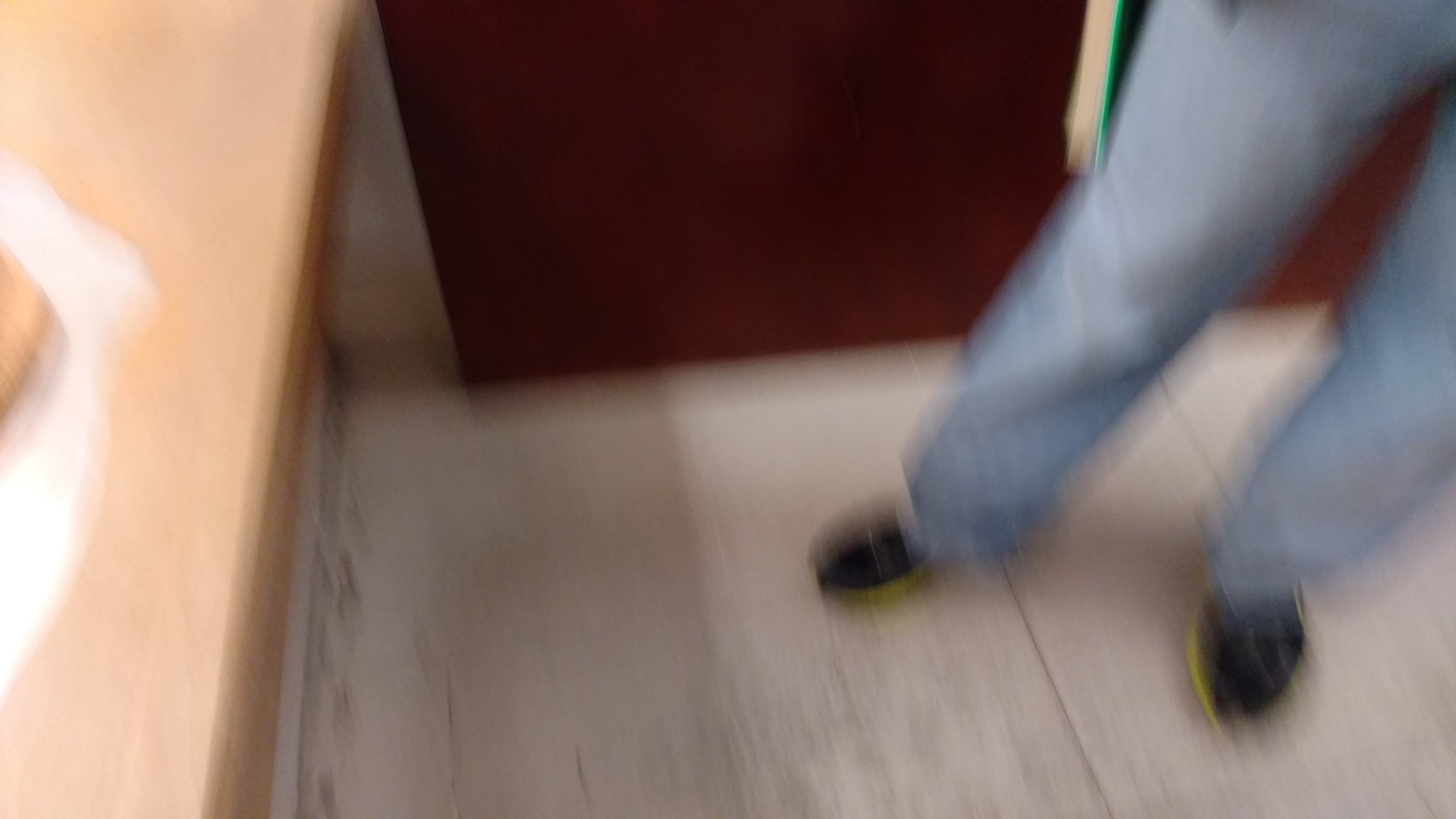The photograph captures a very blurry indoor scene. On the left-hand side, a light brown wooden countertop extends from the top left to the bottom left. A white or light-colored bag seems to be on this shelf. In the middle back of the image, you can see the bottom portion of a dark brown door. The floor appears almost white or very light brown, with possible scuff marks. On the right side, descending from the upper right to the bottom right, is a pair of legs clad in blue jeans and dark-colored, likely black, sport-type sneakers with yellow soles. The jeans cover the top part of the shoes, making it difficult to determine whether they are low-tops or high-tops. Additionally, it seems the person might be holding something with a green outline, possibly paper, though this is hard to confirm due to the blurriness of the image.